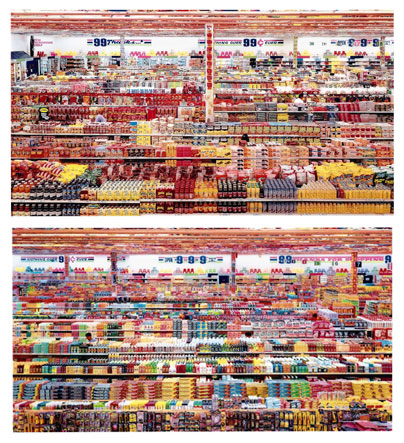This vertical rectangular image appears to depict the inside of a densely stocked store, likely a grocery store. It is divided into two smaller, almost identical rectangles, stacked on top of each other. Each section showcases aisles teeming with various items, creating a palette of vibrant colors: reds, yellows, blues, greens, and more. The upper section features rows of tables laden with products, under a red ceiling, with large windows at the back revealing a glimpse of the sky and distant buildings. The bottom section mirrors this setup, with the same red roofing and windows framing the aisles. Notably, signs displaying the number '9' and '99 cents' can be seen in the background, hinting at price deals. The image is brightly lit, ensuring all details are clear, but no people are visible in the scene.